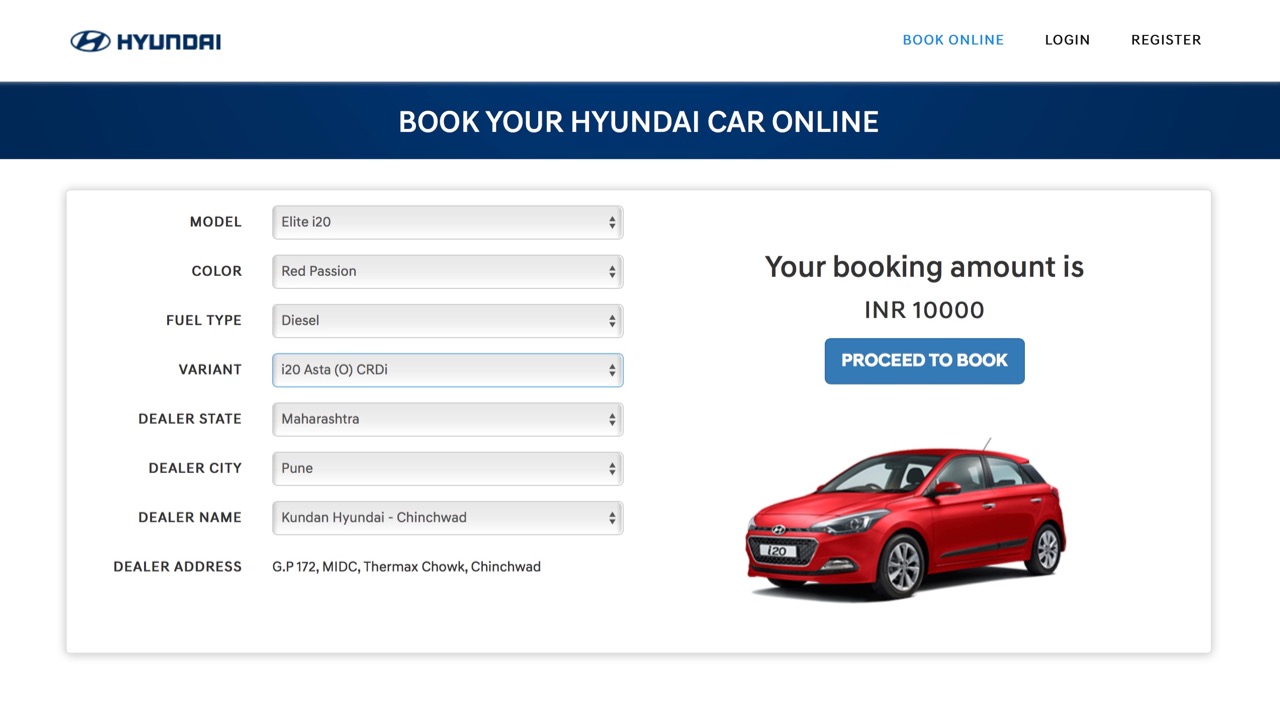This is a screenshot of a desktop browser window displaying the Hyundai website. In the top left corner, the Hyundai logo is prominently featured, consisting of capitalized blue text and a stylized 'H' emblem. The top right corner of the website includes various navigation tools: a blue "Book Online" button, a "Login" button, and a "Register" button. Below this, a blue ribbon banner announces, "Book your Hyundai car online."

The main section below the banner contains numerous fields for detailing the car you'd like to book. The fields, which are all filled out in this screenshot, are as follows: Model, Color, Fuel Type, Variant, Dealer State, Dealer City, Dealer Name, and Dealer Address.

On the right side of the screen, there is an image of a red Hyundai car with a license plate that appears to read "i20." Above the car image, text indicates, "Your booking amount is INR 10,000." Below this information is a blue "PROCEED TO BOOK" button, with the text displayed in capital letters.

The website features a simple, clean design with a navy blue and white color scheme, and ample white space, making it user-friendly and uncluttered.